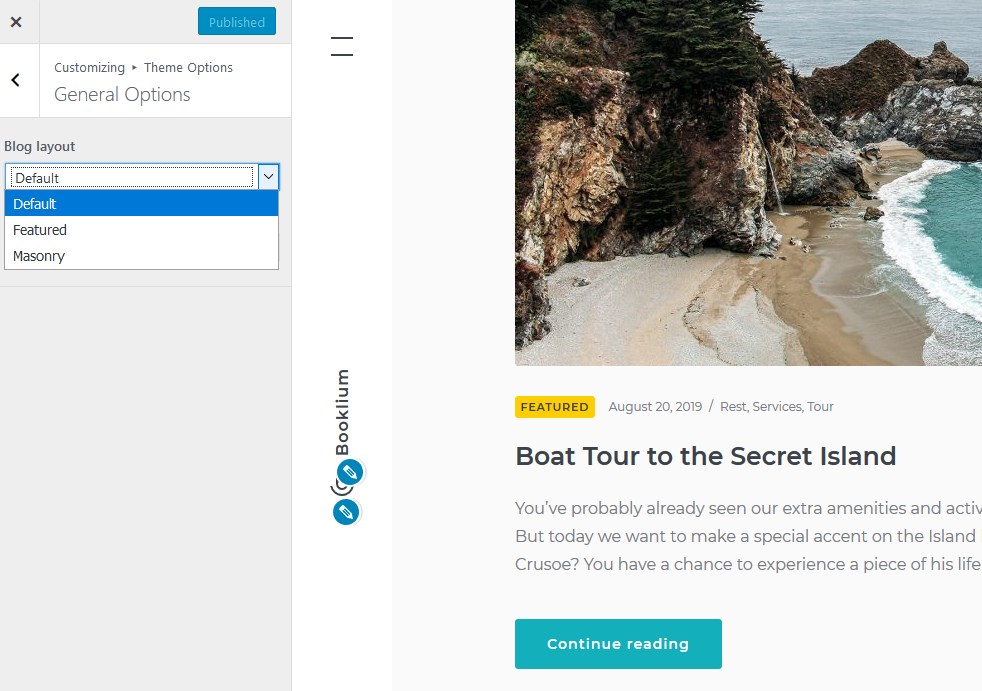The image displays a user interface snapshot featuring a gray horizontal bar on the left side. This bar includes a light blue section extending across it and a blue button labeled "Published." Below this, a white section contains the text "Customizing with the Arrow Theme Options" with a dropdown arrow. Further down, the menu lists "General Options," and below that, "Blog Layout" with a dropdown menu offering choices such as "Default," "Featured," and "Masonry."

On the right side of the image is a picturesque beach scene dominated by a towering cliff. The scene showcases the shoreline, with waves creating white foam as they approach the sandy beach. A yellow square labeled "Featured" appears at the bottom of this scene, followed by the text: "Boat Tour to the Secret Island. You've probably already seen our extra amenities and activities, but today we want to take a special accent on the island. In Crusoe, you have a chance to experience a piece of his life."

Below this description, a blue button prompts viewers to "Continue Reading."